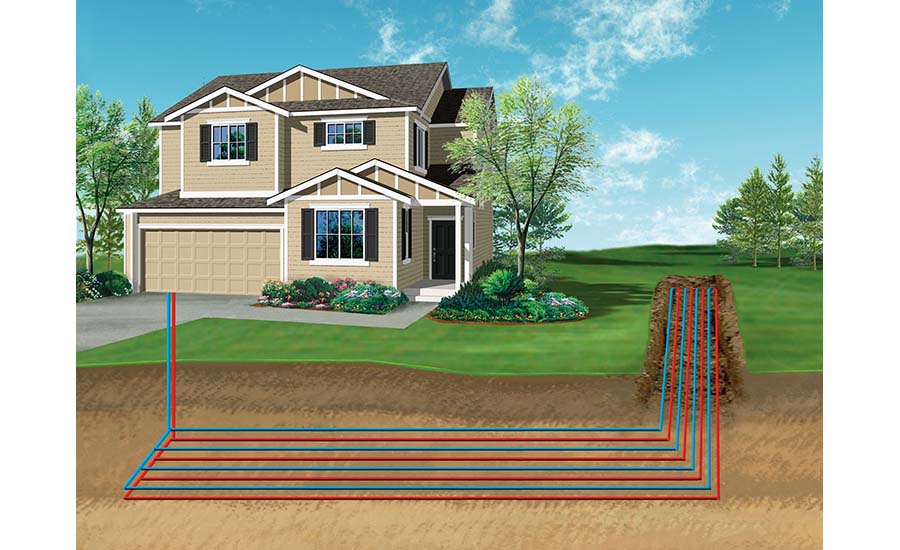The image is a detailed, computer-generated illustration showcasing a modern, beige-colored, two-story residential house situated on the left side. The house features a two-car garage, a brown front door, and white-rimmed windows with brown shutters. The reflection of trees can be seen in the windows. A cement driveway leads up to a covered walkway. In front of the house, to the right of the garage, there is a well-maintained garden full of flowers, including many bushes and roses. Flanking the house are two large trees, and additional trees populate the background under a vibrant blue sky with slight clouds.

The right half of the illustration shows a lush green lawn, contrasting with the brown ground in the front where red and blue underground lines branch out from the house and extend rightward. These lines curve upward at a 90-degree angle and continue off into the distance, representing underground utility installations. The brown coloring around the lines visually distinguishes the underground section from the surface, emphasizing the lines' subterranean nature.